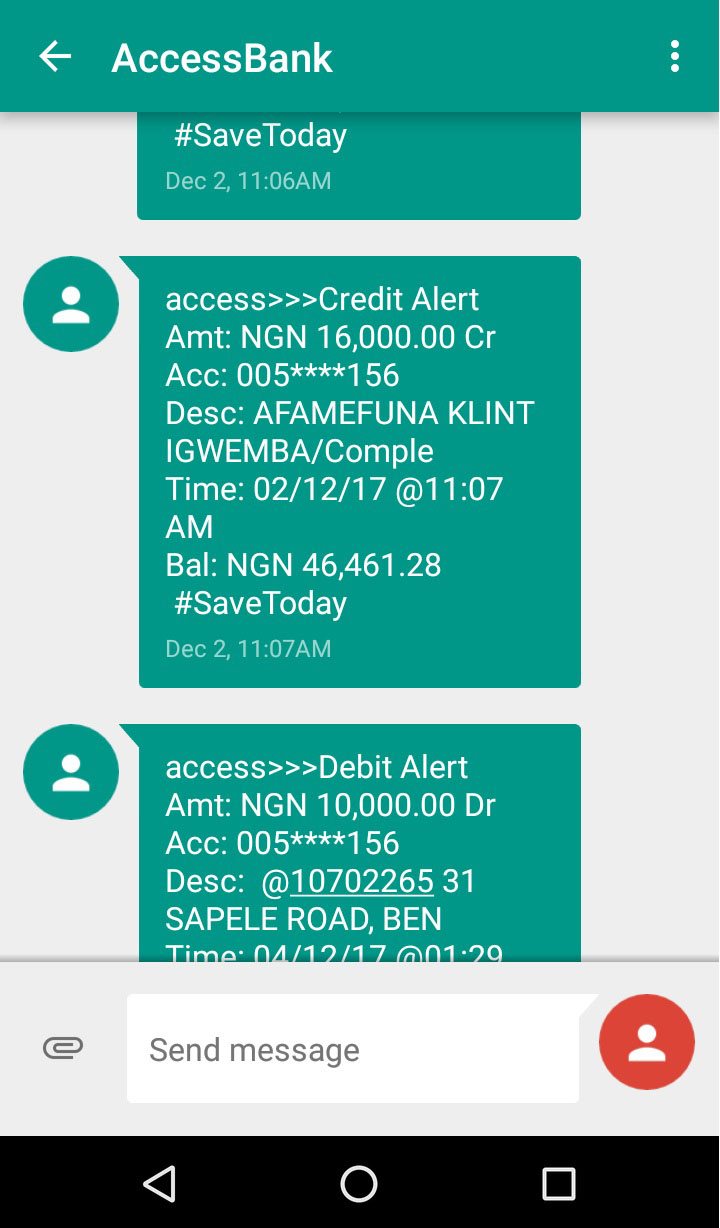A screenshot from a cell phone shows a messaging interface with a green and white top strip. On the left side of the strip, there's a left-facing arrow and the words "Access Bank." On the right side, there are three vertically aligned dots. Below this strip, various messages are displayed, indicating financial transactions.

The first visible message is partially cut off, but it includes the text "#SaveToday December 2, 11:06 AM." The next full message reads: 
"Access →→→ Credit Alert: Amount NGN 16,000.00 CR. Account: ******0156 ESC: AFAMEFUND KLIN TIGW MBA/COMPLETE. Time: 02/12/17 at 11:07 AM. Balance: NGN 46,461.28. #SaveToday December 2, 11:07 AM."

Following this, another message is partially visible and says:
"Access →→→ Debit Alert: Amount NGN 10,000.00. Direct Account: ******0156."

The messages detail recent transactions and updates on the balance of the account associated with Access Bank.